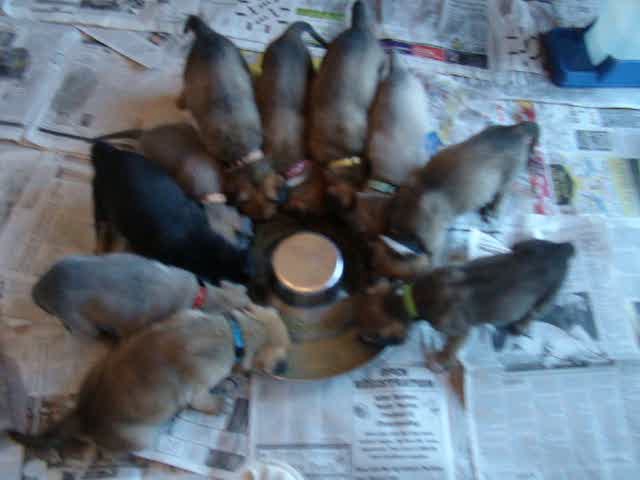This image captures a slightly out of focus, overhead view of a litter of 10 short-haired puppies gathered around a circular, silver metallic feeding bowl or dish, reminiscent of a Bundt pan. They are all intensely focused with their heads down, appearing to be eating or drinking. The puppies' short fur coats vary, with most being light brown and a few dark brown or black, all adorned with collars in various colors such as blue, red, green, white, yellow, and pink. They stand on a floor covered haphazardly with black and white newspaper, which has been unfolded to create a makeshift feeding area. The scene portrays a chaotic yet adorable meal time for the puppies.